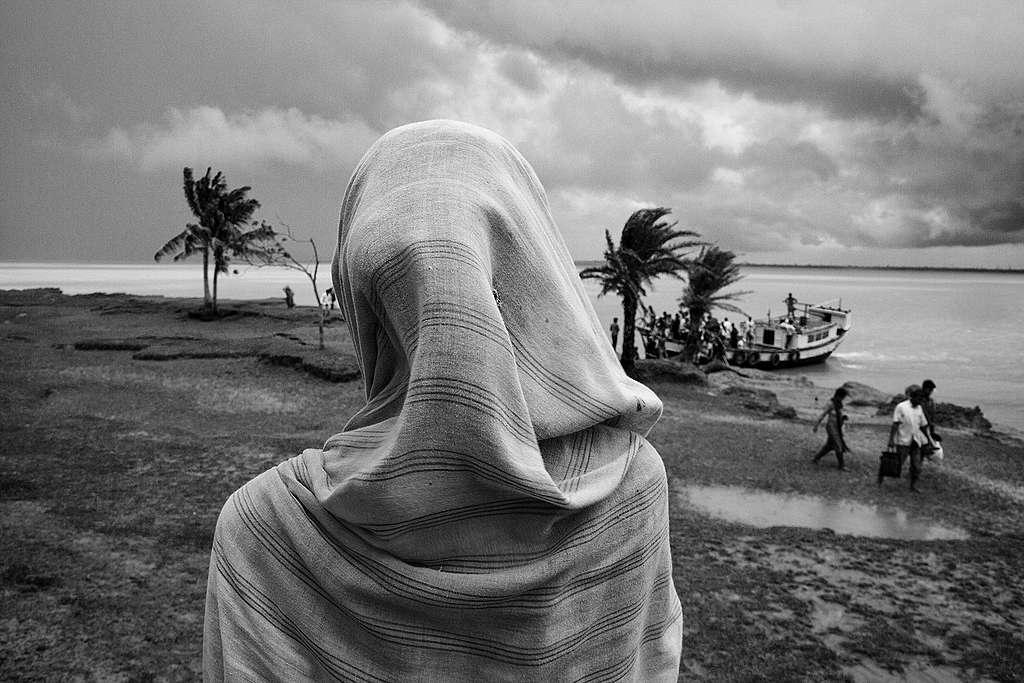In this black and white photograph, a woman stands with her back to the camera, draped in a head covering that also shrouds her shoulders. She gazes out over a water scene, possibly the shore of an ocean or sea. The sky above is filled with stark, dark clouds, suggesting an impending storm. To both the left and right of her, there are palm trees swaying in the wind. Off to her right shoulder, a boat is anchored, where multiple people are either boarding or disembarking, some carrying luggage or briefcases. In the foreground and near her right side, small pools of water dot the beach. Further in the distance, three figures—two men and one woman—walk across the shoreline, adding to the somber, atmospheric mood of the scene. The entire landscape, from the grayish waterway to the overcast sky and the shadowy beach, conveys a monochromatic palette that heightens the photo's dramatic and contemplative tone.